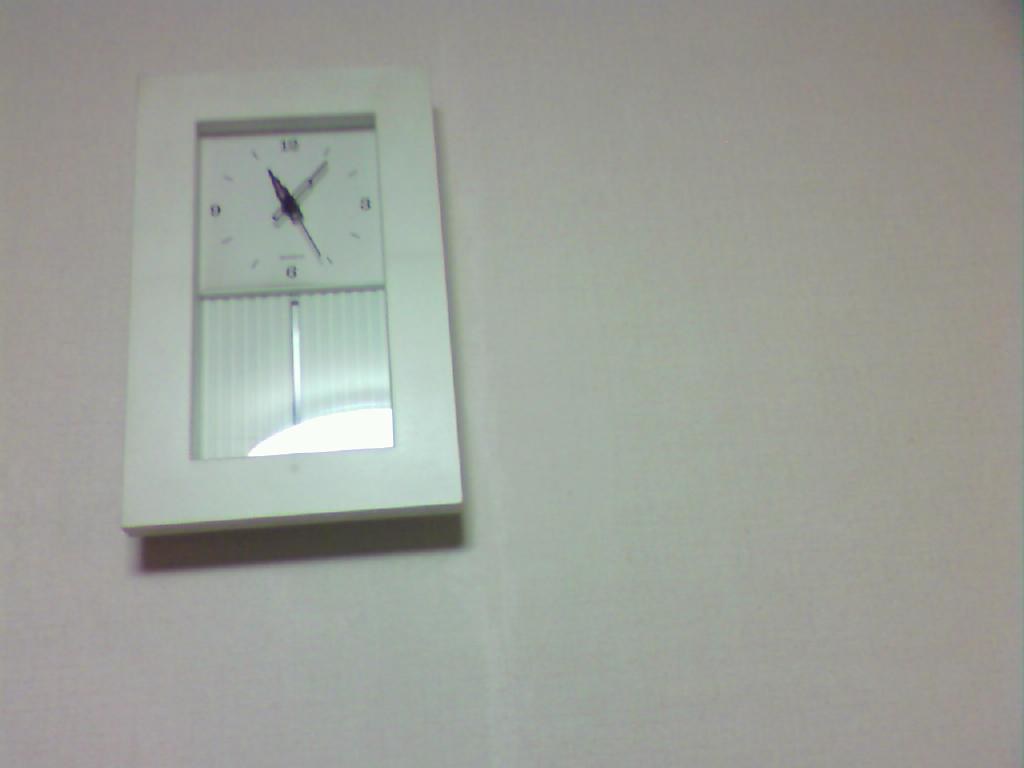Here is a refined and detailed caption for the image:

"A rectangular wall clock with a thick white frame hangs vertically against a white wall. The clock face is predominantly white, featuring bold black hour and minute hands. The numerals 2, 3, 6, and 9 are distinctly visible, while the other hours are marked with notches. The lower half of the clock face has a textured white area with subtle grooves. A slender metal rod extends into the middle of the clock, which adds a slight metallic sheen. Light reflects gently off the bottom section of the clock face, accentuating its clean, minimalist design. The wall clock casts a faint shadow on the wall behind it, enhancing the scene with a sense of depth. The overall aesthetic is crisp and modern, complementing the neutral tones of the white wall."